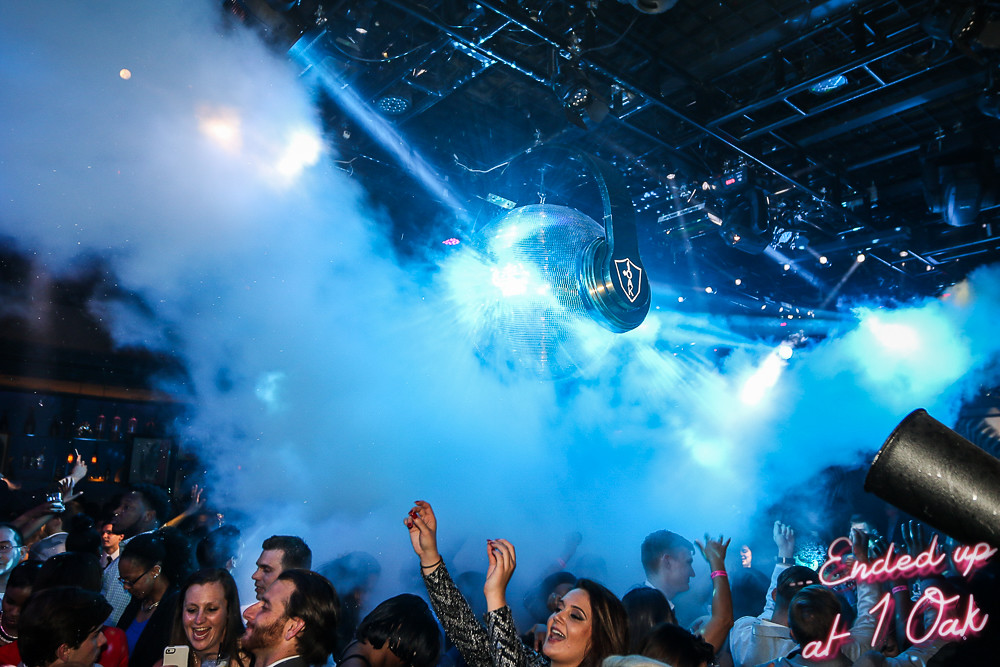The image captures the vibrant atmosphere of a nightclub event at One Oak. At the center of the scene, a massive, shiny blue disco ball adorned with oversized DJ headphones emits a glowing blue light, creating a captivating centerpiece. The crowd below is lively, with many people raising their arms towards the left, likely where the stage is situated. A prominent young woman stands out in the foreground, her hands lifted high and adorned with red-painted nails. She has dark hair and wears eye-catching black and silver attire, complemented by dark red lipstick. The setting is filled with smoke and the blue strobe light enhances the club’s dark, warehouse-like environment. Above the crowd, an intricate trellis adds to the overall ambiance. The phrase "Ended Up At One Oak" is prominently displayed in the lower right corner, marking the image with a distinctive watermark.